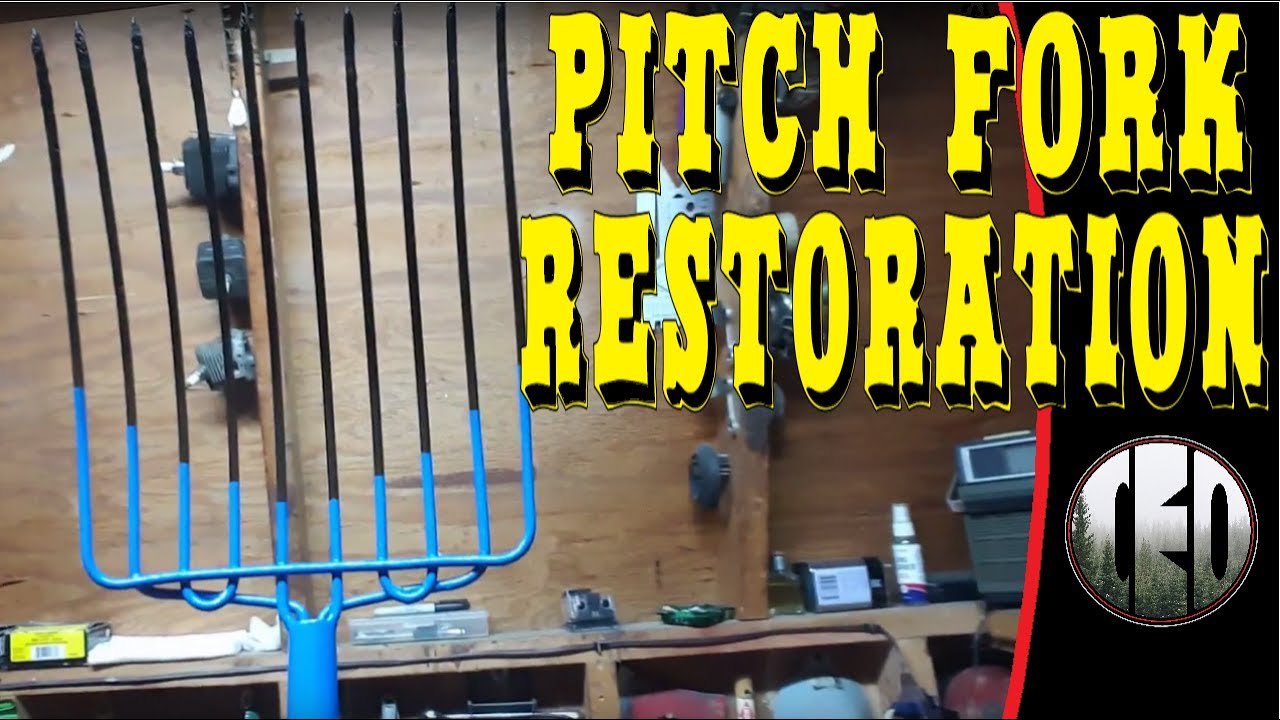The image prominently features large yellow text in the upper right corner that reads "PITCHFORK RESTORATION" in an all-cap font. Directly below this text is a circular logo labeled "CEO" in white, overlaid on a forest scene with trees. A thin red line runs vertically along the right edge of the image. The majority of the visual space is occupied by a central and left-side image of a blue pitchfork with black-tipped prongs, set against a rustic wooden wall. The wall is adorned with various tools and objects, including items like a pencil sharpener, telephone, glue, dropper, medicine, a Sharpie, and a measuring tape, making it appear like a well-equipped workspace or garage. The pitchfork, with its modern light blue handle and restored aesthetic, suggests a blend of old and new against a backdrop of practical tools.